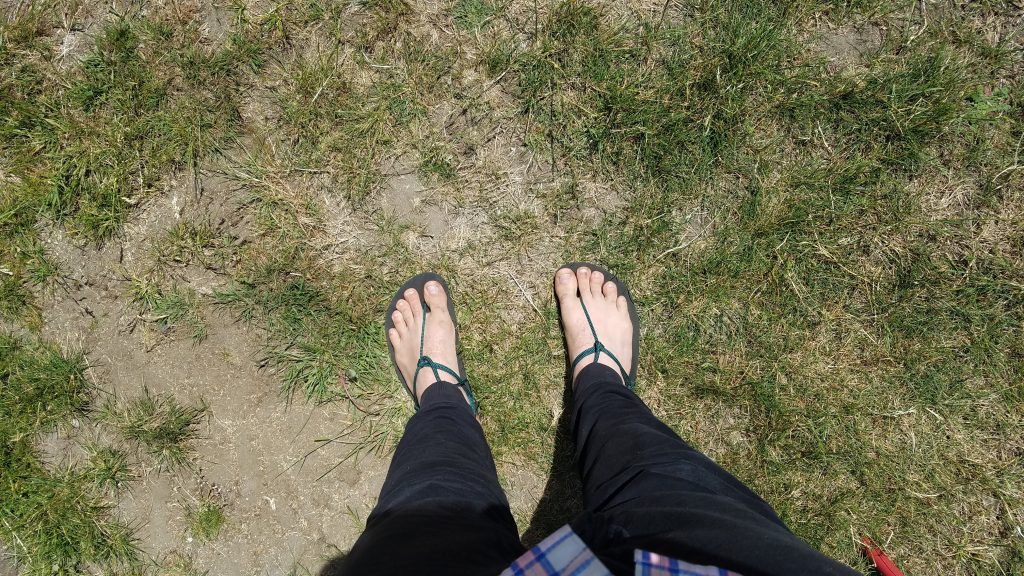In the photograph, we see a close-up of an individual's feet adorned in grey sandals. The sandals are designed with thin green straps that weave between the big toe and encircle the base of the foot. The person is dressed in black pants, paired with a shirt that features horizontal stripes in grey, blue, and pink hues. 

In the background, the ground appears dry and parched, characterized by a rugged, brown terrain. Scattered across this arid landscape, various lengths of grass blades and weeds are visible, with some patches of grass appearing longer than others. The scene conveys a sense of neglect and harsh environmental conditions.